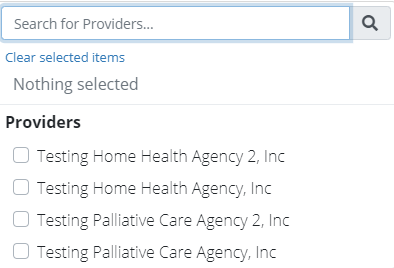The image displays a user interface with a white background. At the top of the interface, there is a light blue box containing another blue box. Within this nested blue box, the text reads "Search for Providers." Directly below, there are options labeled "Clear Selected Items" and "Nothing Selected," followed by a horizontal line that separates these options from the list below.

The list is titled "Providers" and features four selectable options, each accompanied by a checkbox. The providers included are:

1. Testing Home Health Agency 2 Incorporated
2. Testing Home Health Agency Incorporated
3. Testing Palliative Care Agency 2 Incorporated
4. Testing Palliative Care Agency Incorporated

Each provider's name is prefixed with a checkbox, allowing users to select or deselect items as needed. The design is clean and functional, focusing on the task of selecting healthcare providers.